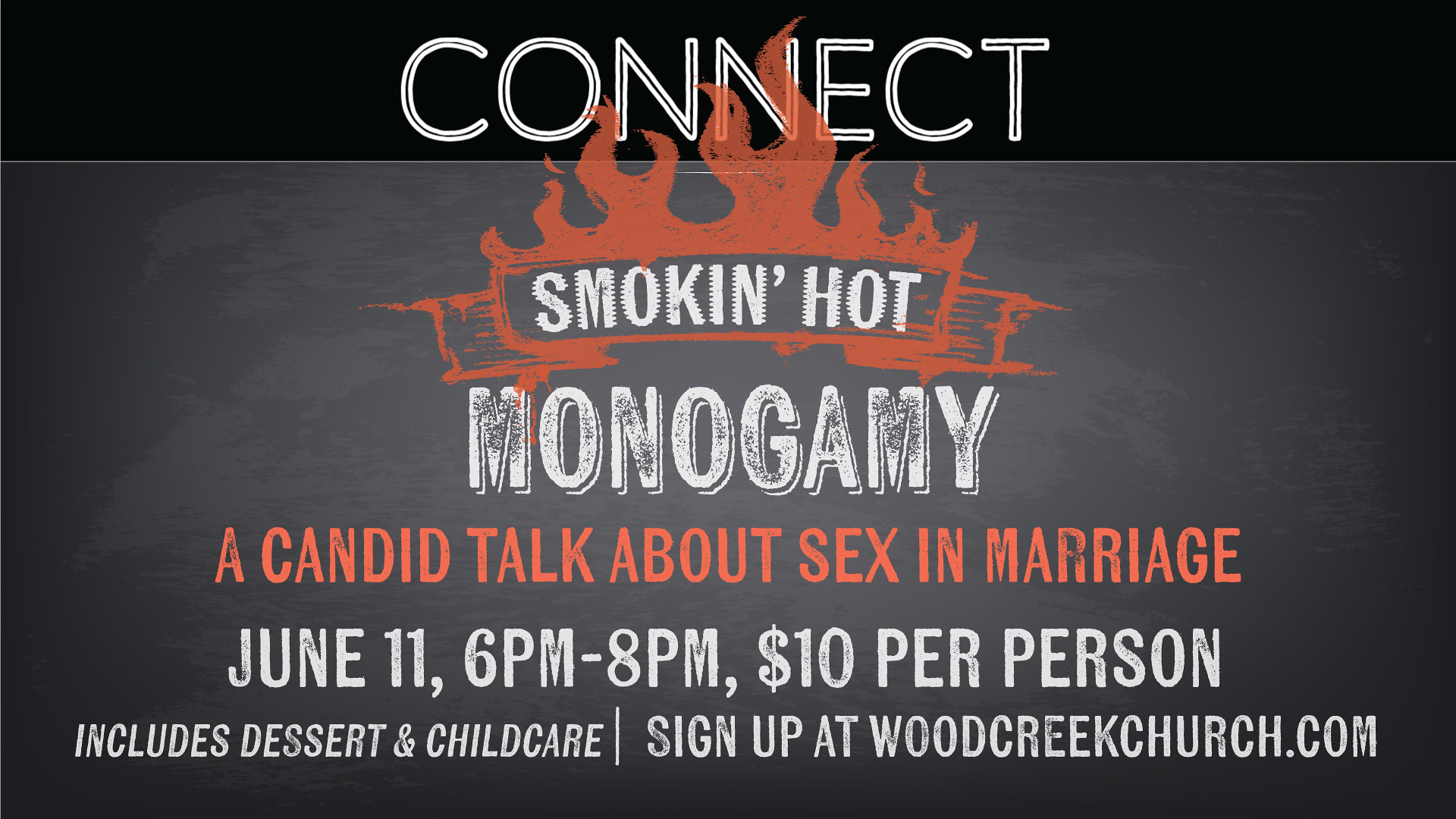The advertisement poster features a striking black background with a prominent white banner at the very top that reads "Connect." Below this, there's a slightly lighter black section with a gray film overlay, giving it a digital chalkboard appearance. The central feature of the design is a dramatic logo that reads "Smokin' Hot" in bold white letters, enclosed in an orange banner and surrounded by vibrant flames. Below the logo, "Monogamy" is displayed in large, bold white letters. Following this, an orange text line reads "A candid talk about sex and marriage." Further details are provided in smaller white text, including the event date and time: "June 11, 6 p.m. to 8 p.m." and cost: "$10 per person," specifying that the price includes dessert and child care. The poster concludes with a call to action in smaller text at the bottom, "Sign up at woodcreekchurch.com." The primary colors used throughout the design are black, white, and orange, creating a visually striking and cohesive look.